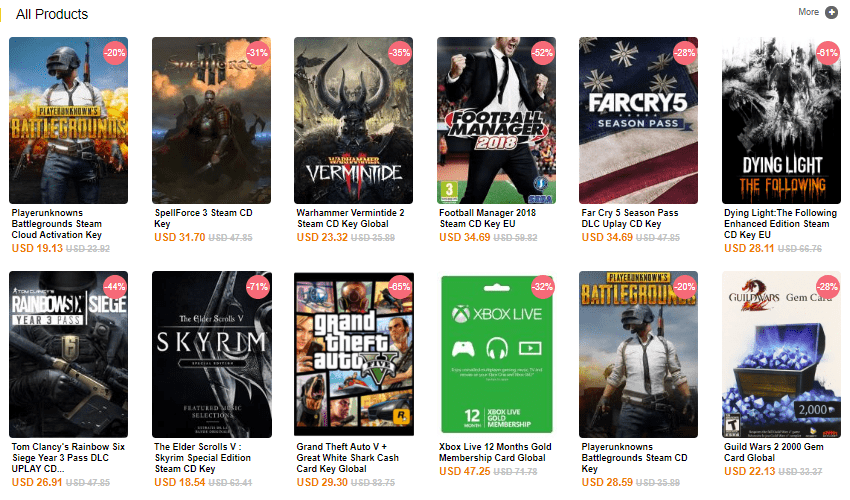In the upper left corner, the phrase "All Products" is displayed in black, followed by a thin yellow line. On the far right, there is a gray section with the word "More" contained in a circle with a white plus sign in the center. 

Beneath this, a series of video game covers are shown. In the top left, "PlayerUnknown's Battlegrounds Steam Cloud Activation Key" is labeled in black text, priced at USD 19.13 with the original price of USD 39.12 grayed out and crossed through. Below, each game has its current price highlighted in yellow, with the original prices grayed out and struck through to indicate discounts. 

The names of the games, also displayed in black, include "SpellForce 3 Steam CD Key" priced at USD 31.70 (originally USD 47.85), followed by titles such as "Warhammer," "Football Manager," "Far Cry 5 Season Pass," "Dying Light," "Tom Clancy's," "The Elder Scrolls V," and "Grand Theft Auto V." Additionally, there is an "Xbox Live 12 Months Gold Membership," "PlayerUnknown's," and "Guild Wars 2." 

The layout has six game covers on the top row and six on the bottom row. Various colors, including red, white, blue, and green, decorate the layout. Each game cover features a small red circle in the top right corner marking the discount percentage, such as 28%, 20%, 35%, and 52%.